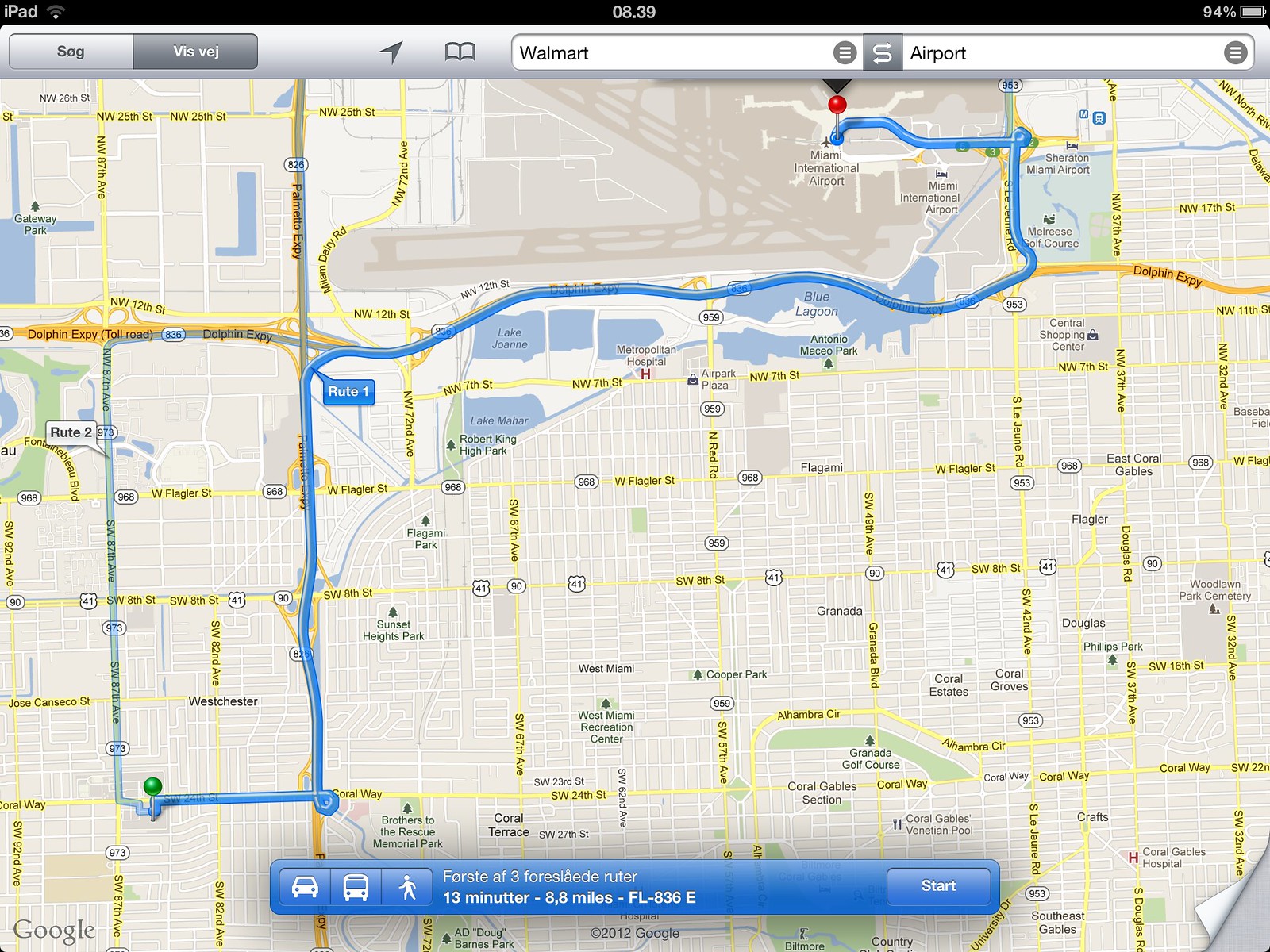This image depicts a navigation map displayed on an iPad screen. The top of the screen shows the device status, with the time marked as 8:39. The map is set to guide the user to Miami International Airport, shown as the endpoint. A blue line indicates the route, starting from a location marked by a green pin. 

In the search bar at the top, "Walmart" is listed as a previous search, and "airport" is the current destination search term. The map displays the total journey as 13 minutes and 8.8 miles. A prominent "Start" button at the bottom signals the initiation of route guidance.

Additionally, the iPad's battery status is depicted, showing 94% remaining. An icon in the bottom right corner suggests an interactive element, possibly for scrolling or turning pages within the application. There appears to be an acronym or text "S-O-G-V-I-S-V-E-G" that might be in another language, adding a layer of complexity or context-specific detail to the image.